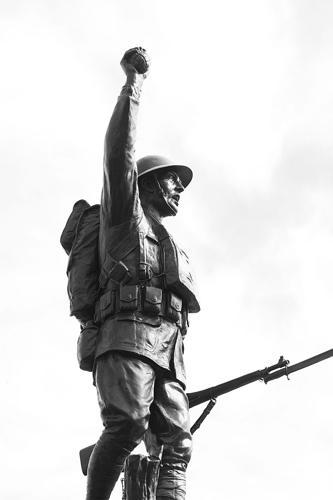The image is a black and white, vertically rectangular photograph without a border, featuring a gray, almost black, statue of a WWI era infantryman soldier. The soldier is facing the right and is portrayed in full military uniform, complete with a round-shaped helmet, a belt with numerous small pockets, and a backpack. The soldier's right arm is raised high above his head, clutching a hand grenade, while his left hand holds a long rifle with a bayonet fixed at its tip, down at his side. Additionally, there is a bag positioned in front of his chest and another one between his legs. The background of the image depicts a gray sky with white clouds, further emphasizing the statue's dramatic stance. The sunlight illuminates the front and face of the soldier, who appears to be screaming, capturing a moment of intensity and determination.